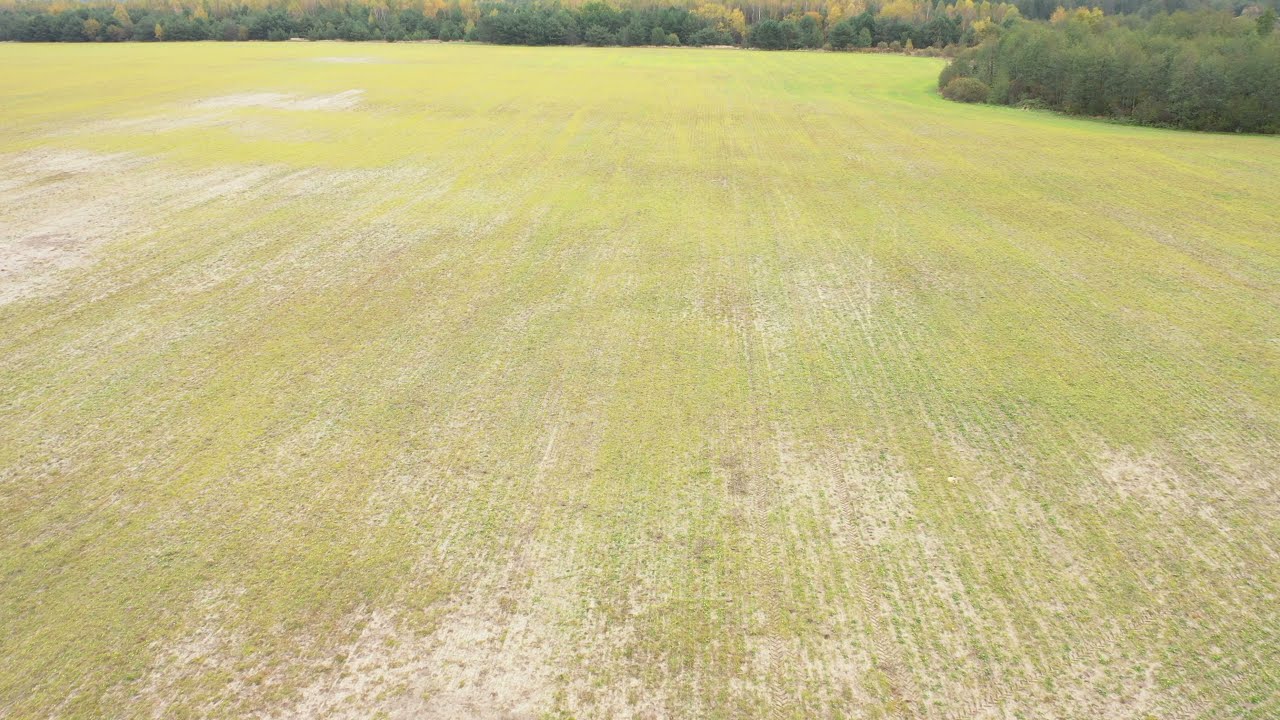This photograph, oriented as a horizontal rectangle, captures a vast, open field from a slightly elevated perspective. The field is a mix of greens, browns, beiges, and grays, indicating a blend of grassy areas with bald patches of dirt and gravel, especially noticeable in the middle to lower parts and the upper left corner of the image. In the distant background, occupying the upper sixteenth of the photo, is a continuous line of trees spanning from left to right, with a denser cluster in the upper right corner. The trees predominantly display shades of green, though some lighter green foliage suggests the early stages of color change. This outdoor scene, devoid of any people, vehicles, buildings, or text, is richly detailed yet serene, and it is clearly captured during daylight hours.